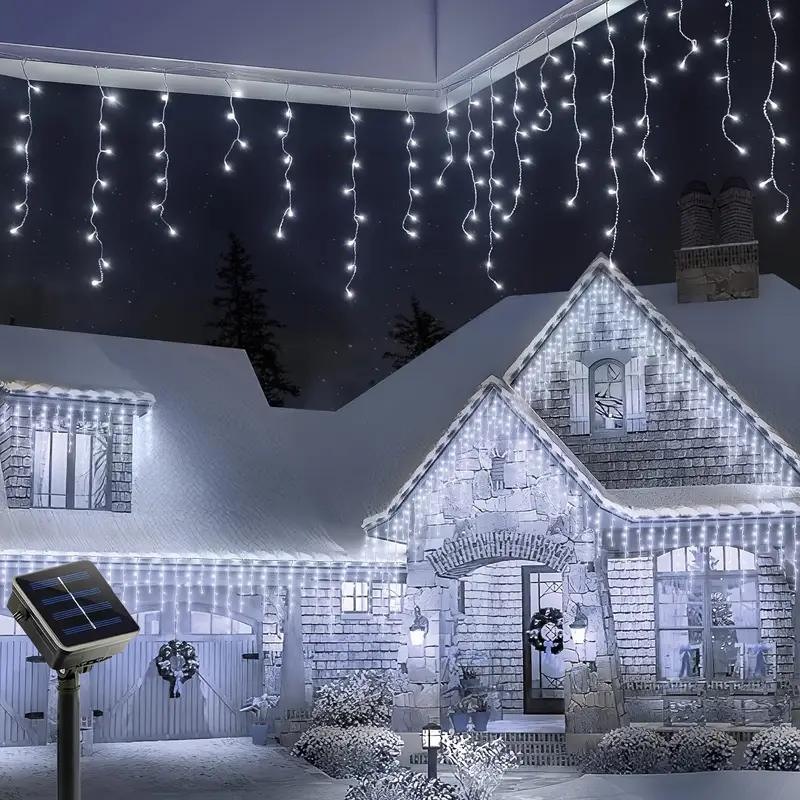This is a captivating nighttime winter scene of a two-level house adorned for Christmas. The house, clad in light gray siding, is blanketed in snow from the roof down to the walkway and front yard. The roof, which features a triangle window surrounded by wood shutters, is festooned with white twinkle lights that hang like icicles. The house gleams from an array of Christmas decorations, including lights outlining the eaves, garage, and windows, as well as a large, beautifully lit Christmas tree visible through the front window. A Christmas wreath with a white bow adorns the garage door, while another festive wreath graces the front door. The porch lights and Christmas lights illuminate the snow-covered bushes and the planters on the front stoop, creating a warm and inviting ambiance. In the background, tall evergreen trees stand against a dark, star-studded sky. However, the scene is slightly marred by a solar power unit in the bottom left corner, which distracts from the otherwise picturesque view.